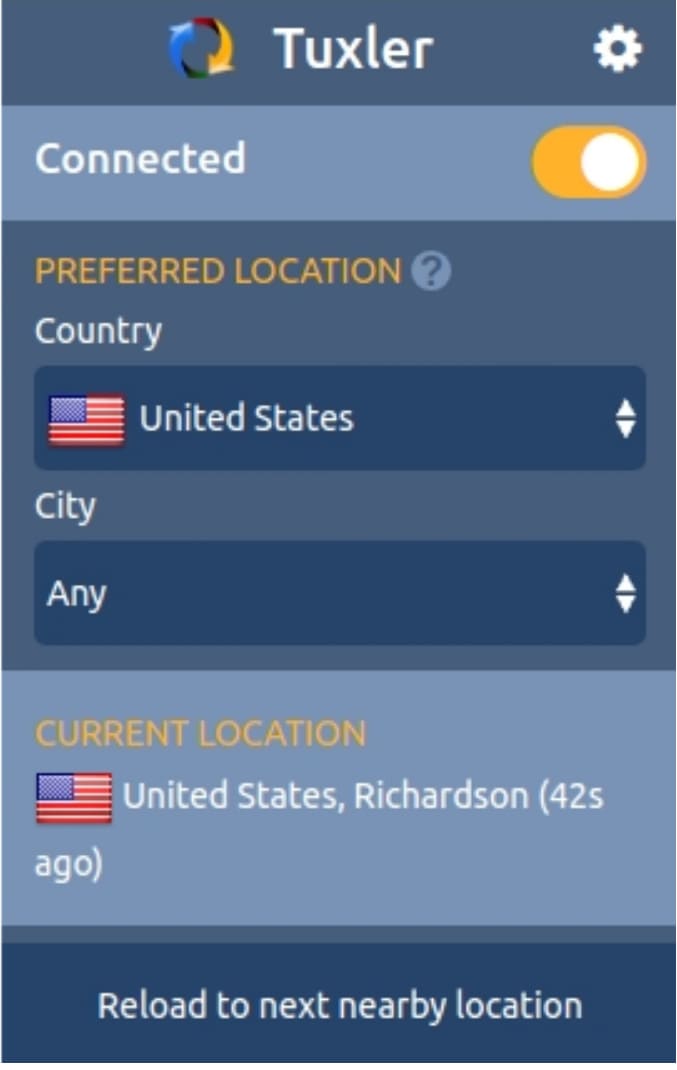The image is a screenshot of the Tuxler app interface, prominently displaying the app's brand icon on the left. The word "Tuxler" is spelled out in white beneath the icon. Directly below, the status "Connected" is indicated, set against a light gray background. Adjacent to this, on the right side, is an oval toggle switch featuring a white circle positioned to the right, signifying that the connection is currently active.

Below this status section, "Preferred Location" is highlighted in yellow. The subsequent section titled "Country" shows a drop-down menu, marked by a box with dual arrows pointing up and down. This box currently displays the United States flag, signifying that the United States is selected. Immediately beside it, the label "United States" is clear, although users have the option to select any country available within the menu.

Next, the "City" section presents another drop-down box set to "Any," allowing users the flexibility to choose any city they prefer. The current location is denoted by an American flag adorned in red, white, and blue, specifying "United States, Richardson." This information is time-stamped as "42 seconds ago," enclosed within brackets and displayed in white text over a light gray background.

Finally, beneath this information, there is an option labeled "Reload to Next Nearby Location," set against a darker gray background. This function suggests that the app is likely a VPN service, providing users the ability to select and switch their virtual location to various cities and countries as available within the app's offerings.